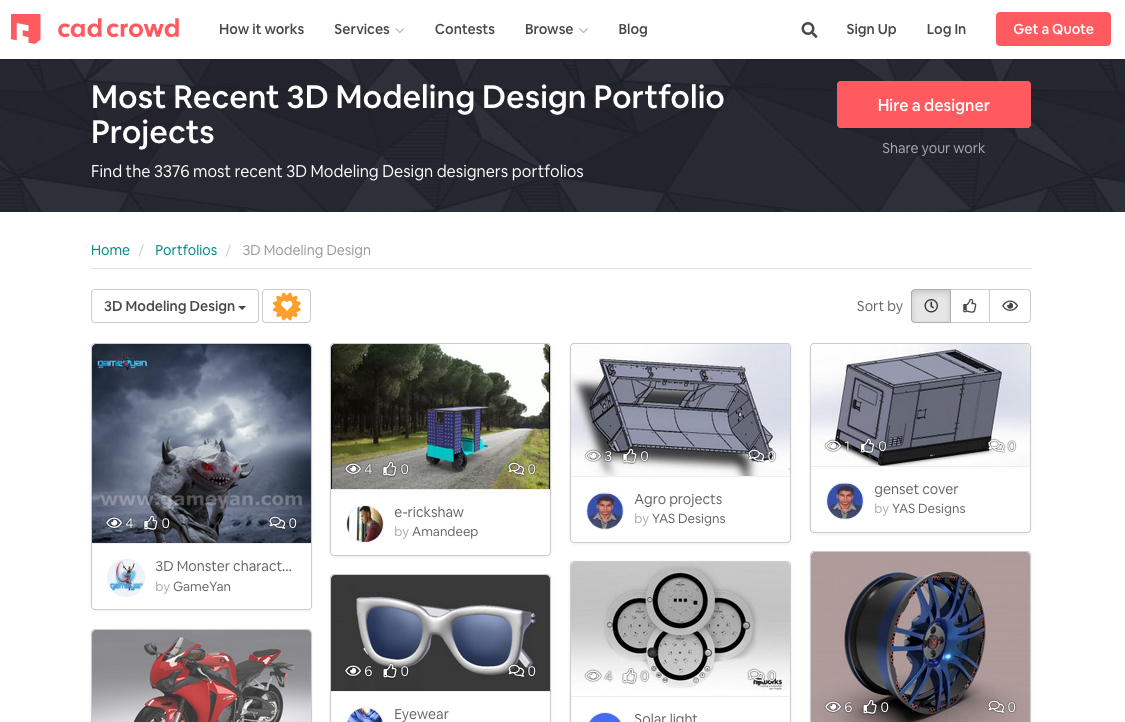The image depicts a webpage from CADCROWD. In the top left corner, the site name "CADCROWD" is prominently displayed in red print. Adjacent to it, in smaller black text, are the navigation links: "How It Works," "Services," "Contests," "Browse," and "Blog." Further to the right, there's a black magnifying glass icon labeled "Further Search." Next to this, the options "Sign Up," "Log In," and "Create or Get a Quote" are presented in white text on a red background. 

Below the navigation bar, a black banner with white text reads: "Most Recent 3D Modeling Design Portfolio Projects. Find the 3,376 Most Recent 3D Modeling Designers Portfolios." On the right side of this banner, a red tab with white text says "Hire a Designer," and underneath it is the option "Share Your Work."

The main background transitions to white, and there is a breadcrumb trail that reads "Home / Portfolios / 3D Modeling Design" with "Home" and "Portfolios" in teal blue-green text. Underneath, there is a header "3D Modeling" with an associated drop-down menu. The content is organized in a grid format, displaying four categories across the top row and four more underneath, offering different sections to explore.